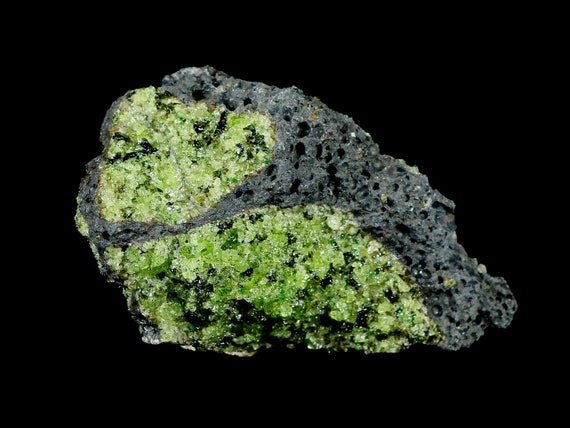This photograph showcases a geode positioned against a stark black background. The geode is split open, revealing its intricate interior. On the left side, the surface features a bumpy, crystalline pattern in various shades of green reminiscent of green tea, with small flecks of dark and light gray. The texture is rugged and rock-like, with numerous tiny projections. On the right side, the geode's exterior is predominantly dark gray, pitted, and mottled, with some white sections. The split reveals an inner structure where greenish crystals dominate, separated by a thin line of gray. The green crystals display a gradient from light green to dark green, including some clear white bits. The entire object, though unlabelled and unsigned, presents a striking contrast between its vibrant, crystalline interior and its rough, earthy exterior.